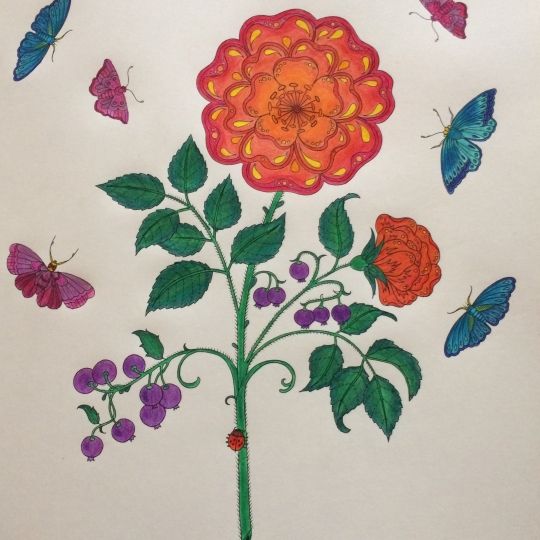The image is slightly taller than it is wide, bordering on a square aspect ratio. It appears to be a finely detailed artwork, possibly created using needlepoint, colored pencils, or delicate watercolor techniques. At the center of the image is a green stem, upon which a red ladybug is seen climbing. The main stem sprouts several offshoots, including branches that bear purple berries, and three additional stems adorned with leaves. There are also two striking orange flowers blooming from the main stem.

Adding to this picturesque scene, there are three blue butterflies flitting about; two on the right-hand side and one in the upper left corner of the composition. Complementing these are three multi-hued butterflies with predominantly purplish-magenta tones—one located in the upper right and the remaining two on the left-hand side, adjacent to the flower.

The entire scene is set against a background that resembles artistic paper, imparting a textured, handcrafted aesthetic to the image.